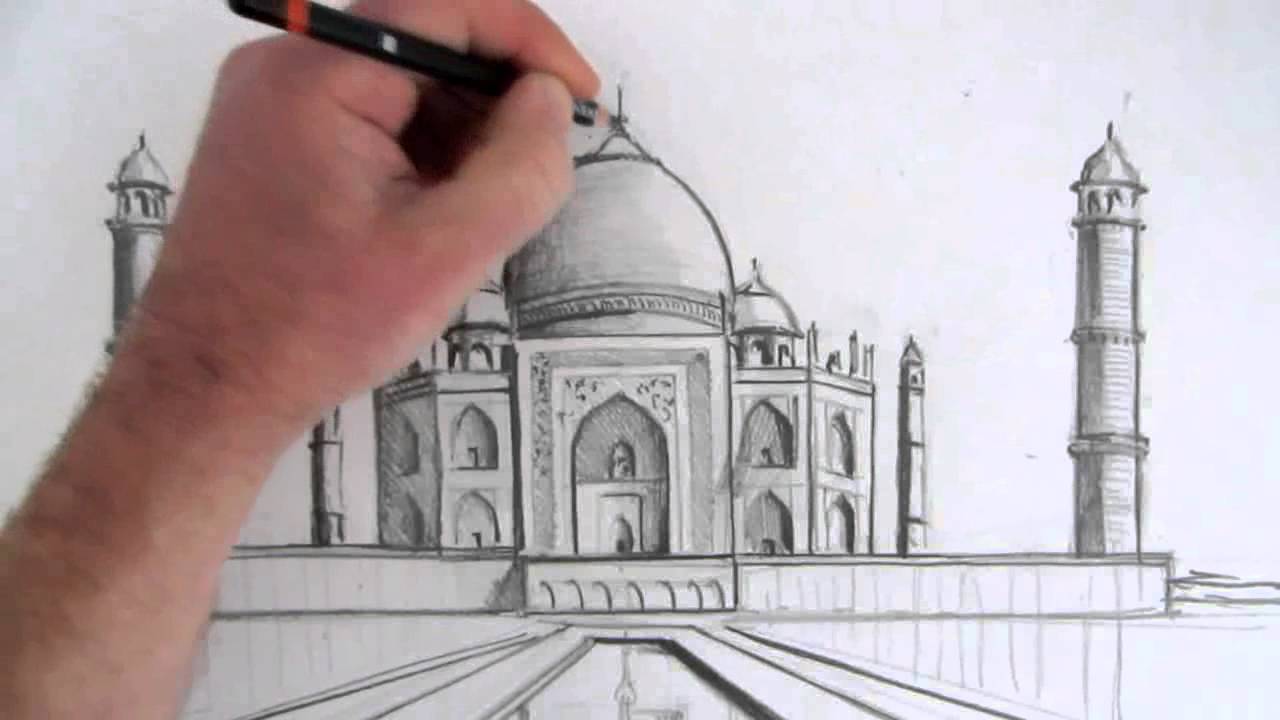The image depicts a detailed drawing of the Taj Mahal being created by a person whose hand is visible in the lower left corner. The artist is holding a black pencil with a red stripe near the bottom, suggesting it is a colored pencil without an eraser. The drawing is done in black and white on a white piece of paper, and the Taj Mahal is illustrated with remarkable precision, including its characteristic domes, minarets, and reflecting pool in front. The picture captures the artist finishing the top section of the Taj Mahal, which features a cylindrical dome. There are architectural spires on both sides, each topped with bell-like structures. Additionally, there's a representation of waterwaves to the right, adding depth to the scene. This intricate artwork, showcasing India's iconic monument built by Shah Jahan in Agra, highlights exquisite attention to detail and artistic skill.